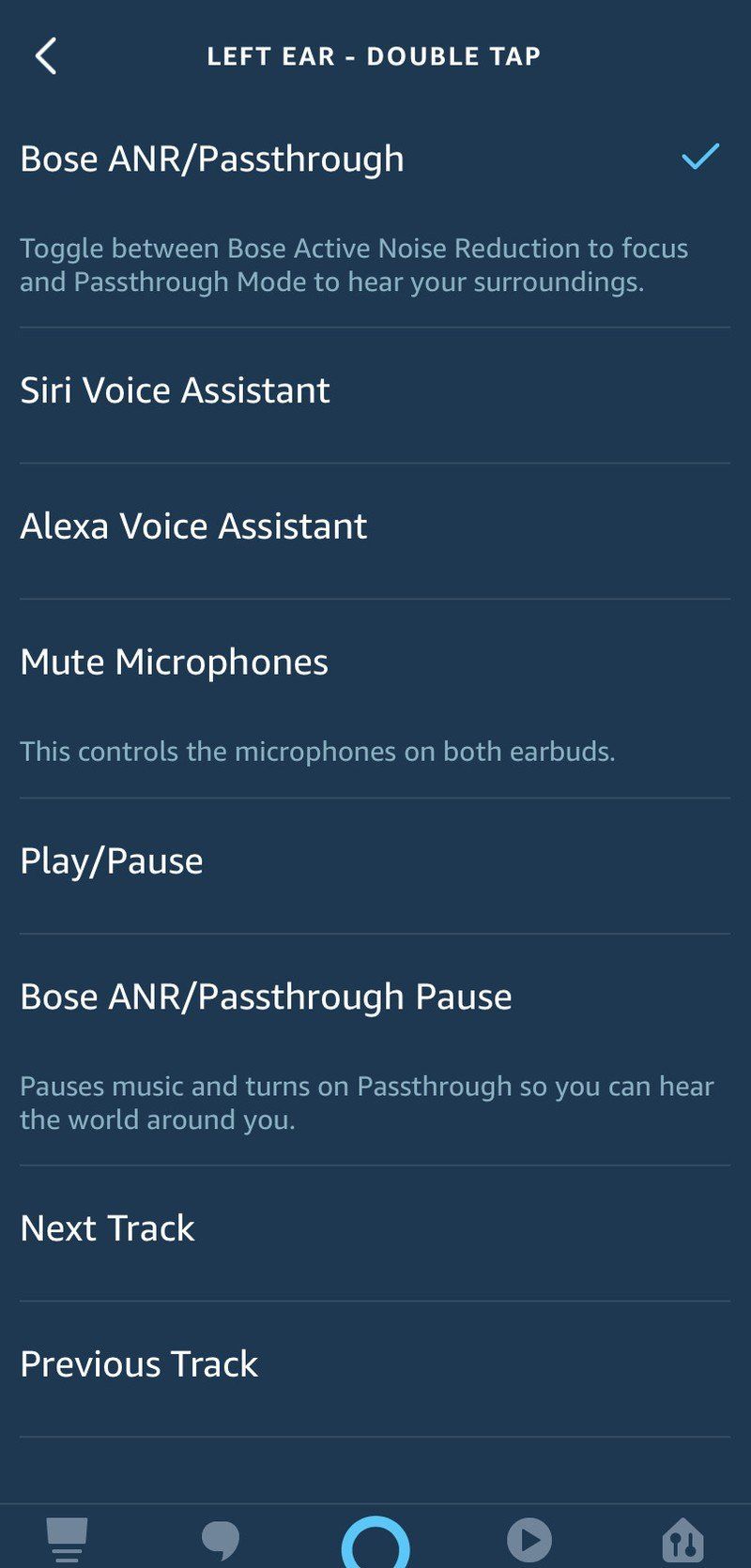The image resembles a settings interface typically seen on a smartphone, displayed against a blue backdrop with white and light blue text. 

In the upper left-hand corner, there's a white arrow tip pointing left. Centered on the page is the text "Left Ear - Double Tap," followed by "Bose (BO/A forward slash) Pass Through" to the right, accompanied by a light blue checkmark. Beneath that, in light blue text, it says, "Toggle between Bose Active Noise Reduction to focus and pass through mode to hear your surroundings." 

The following sections are listed below in white text:
- "Siri Voice Assistant"
- "Alexa Voice Assistant"
- "Mute Microphones"

Under the "Mute Microphones" section, light blue text states, "This controls the microphones on both of the earbuds."

Continuing in white text:
- "Play/Pause"
- "Bose A/R/Pass Through" with the note in light blue, "Pauses music and turns on pass-through so you can hear the world around you."
- "Next Track"
- "Previous Track"

At the bottom of the image are several icons in a light grayish color:
- A paintbrush icon on the left
- A speech bubble or chat icon
- A light blue circle with a matching blue dot in the middle
- A circle containing a triangle, resembling a play symbol
- An icon resembling a house with two blue symbols inside: one as a bubble on top with a line coming out, and another inverted version of the same symbol with the bubble at the bottom.

These details collectively illustrate the various settings and controls available for a pair of Bose earbuds, highlighting options for adjusting noise reduction, controlling voice assistants, and managing playback and track selection.